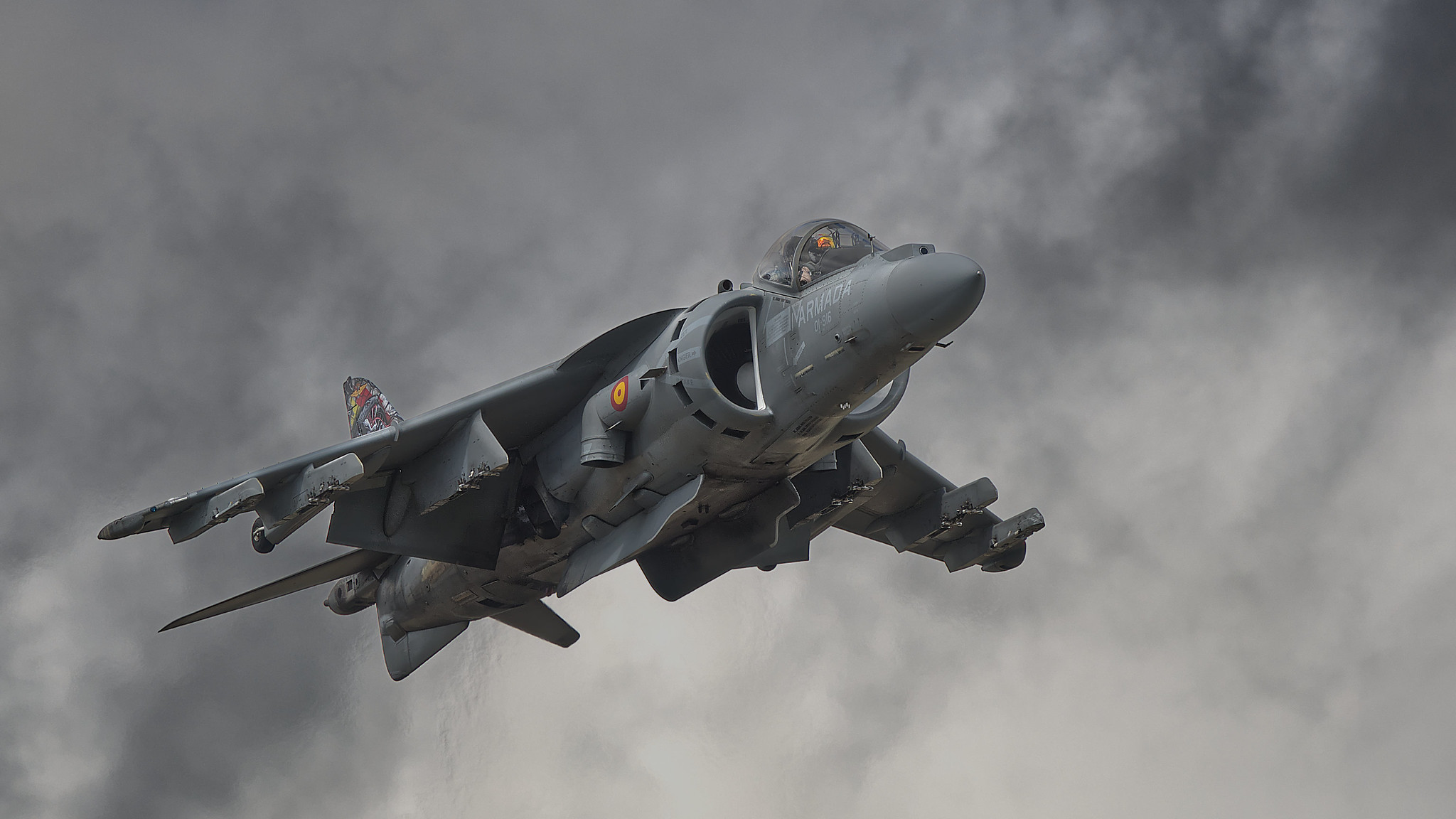This detailed render, possibly from an animation or video game, features a gray fighter jet captured from an aerial, slightly off-angle perspective, emphasizing the underside. The aircraft is set against a very overcast, gray sky, enhancing the overall monochromatic feel of the scene. Notably, there are some identifiers on the jet: white text reading "Marmada" is visible on the side, and there's a bullseye emblem painted on the body. The jet displays signs of wear and tear, particularly beneath the missile holders which appear burnt or dirty, and the tail fin is marked with graffiti. Additionally, the tail and side carry a white box with gray writing, although the details are too small to decipher clearly. The cockpit reveals a pilot's helmet, providing a subtle yet vital element of color alongside red and orange emblems that possibly signal national or unit affiliation. This image, despite its grayscale appearance, is contrasted by these colorful details, ensuring it cannot be mistaken for an actual photo but rather a detailed and possibly cinematic render.